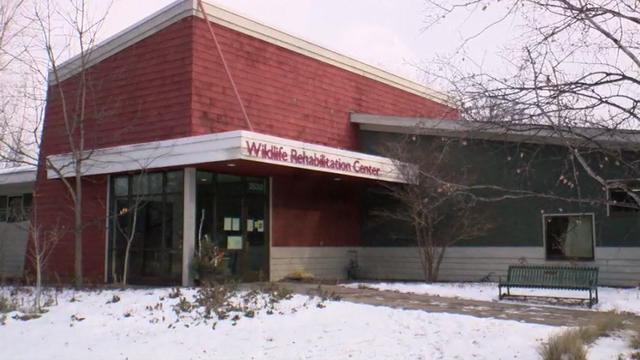The image depicts the exterior of the Wildlife Rehabilitation Center, exhibiting an older photographic quality likely from the 1980s or 1990s. The building prominently features red siding with white trim and is marked by a white awning bearing the red-lettered sign "Wildlife Rehabilitation Center." This section of the building has a square shape and includes a large glass entrance with surrounding windows. To the right of this red-faced portion, there is an attached section with an olive green exterior also trimmed in white. The landscape is coated in snow, indicating a wintry setting. A green bench is positioned in front of a window along a cement walkway. Surrounding the building, there are several bare trees and snow-covered patches of grass, adding to the dreary atmosphere suggested by the gray sky. The scene lacks visible wildlife, reflecting that the center’s activities are likely conducted indoors.